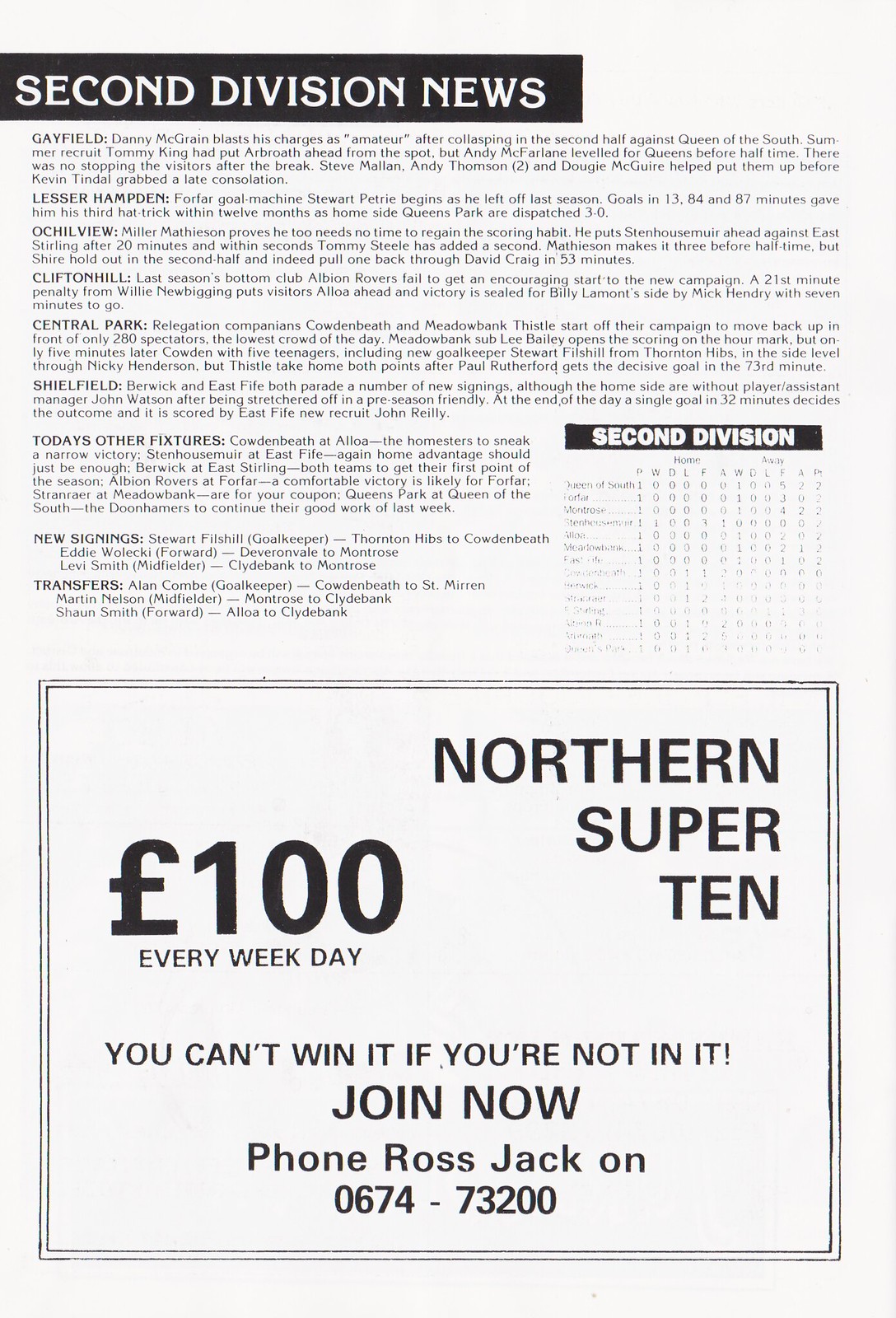This image features a single page from an aged magazine, which occupies the entire frame. The background color is an aged tan, giving a vintage feel. Dominating the top of the page is a black rectangle with the heading "Second Division News" in prominent white letters. The article beneath the headline reports on recent sports events, specifically mentioning "Gayfield", where Danny McGrane collapsed in the second half against Queen of the South after being described as an amateur for blasting charges. Summer recruit Tommy King had initially put their team, presumably Airboats, ahead from a penalty kick, but Andy McFayne equalized for Queen of the South before halftime. The visiting team dominated after the break with contributions from Steve Mellon, Andy Thompson, and Dougie McGuire before Kevin Tindall secured a late consolation goal. 

The lower section of the page contains various texts and sports statistics, including updates on team signings, transfers, home and away games, and scores from teams such as Lesser Hampton, Oakleville, Clifton Hill, and Central Park. To the right of the text, there is a small Second Division chart. At the bottom of the page, there is a neatly outlined advertisement within a square black box, promoting the "Northern Super 10," which offers a prize of 100 pounds every weekday, urging readers to join by contacting Ross Jack at the provided phone number. The text inside the advertisement reads in black: "You can't win it if you're not in it. Join now. Phone Ross Jack on 067473200." The color scheme across the page primarily consists of tan, black, and white, maintaining a consistent and clean presentation.